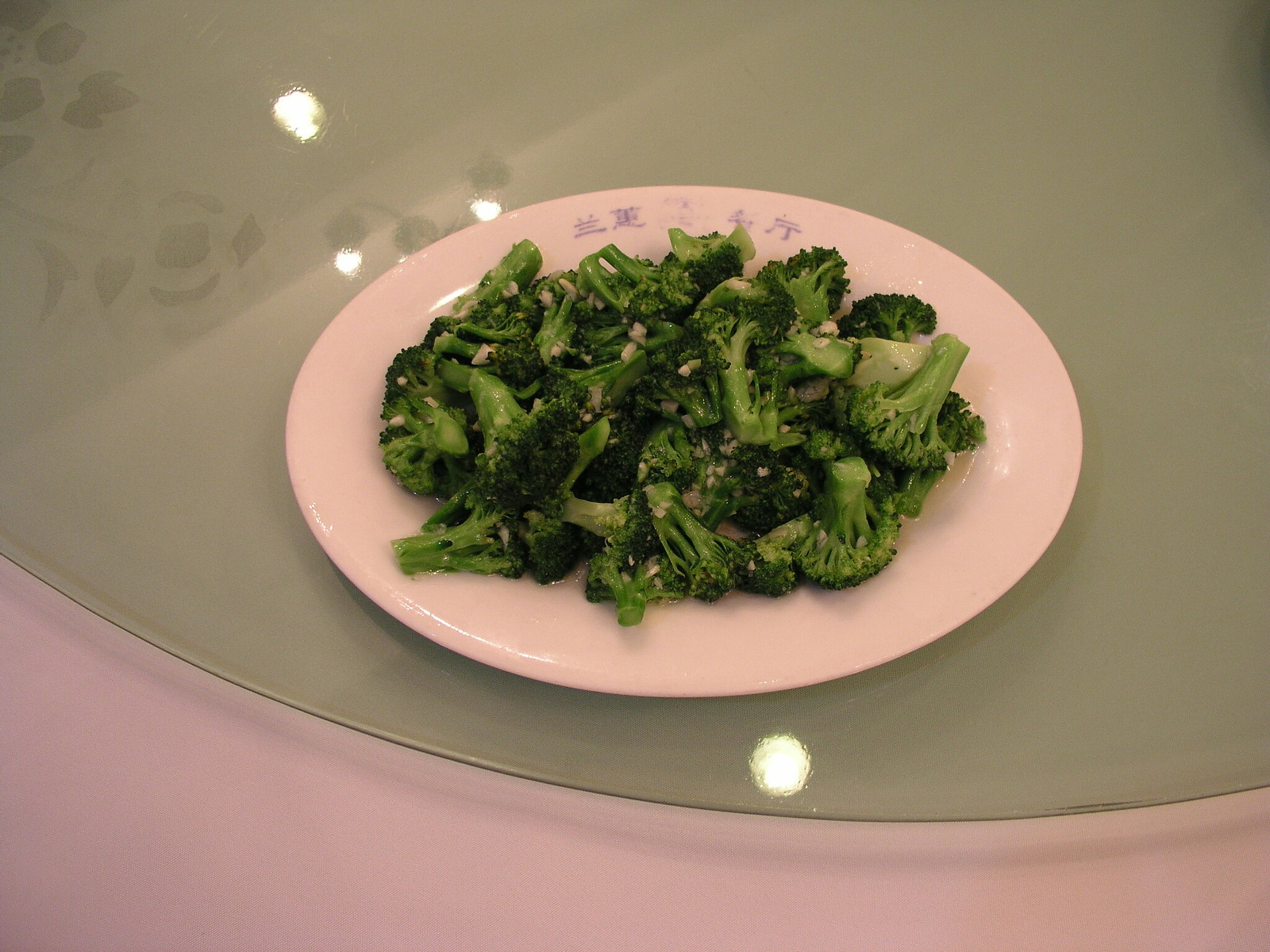The photograph depicts a substantial pile of broccoli, including entire stalks and florets, arranged on a predominantly white ceramic plate adorned with blue or possibly Asian-script characters around its rim. This detailed plate rests atop a glass Lazy Susan, which is a common fixture in dim sum or Chinese restaurants, facilitating easy sharing of dishes. The glass surface of the Lazy Susan features delicate floral etchings and reflects the overhead lighting. The broccoli is interspersed with small, cut-up white pieces of a condiment or seasoning, enhancing its presentation.